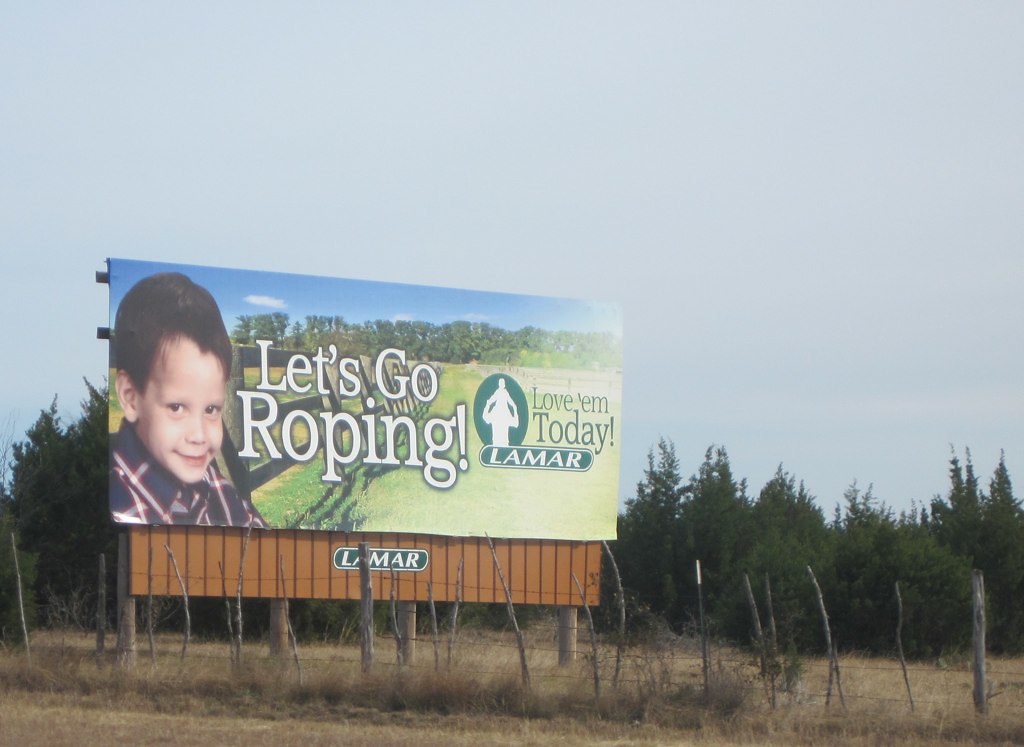This detailed image captures a rural outdoor setting dominated by a large rectangular billboard alongside a roadway. At the forefront of the billboard, a smiling young boy, who seems to be a white child with brown hair, is showcased on the left side. He wears a plaid shirt with a visible collar, adding a touch of realism to the scene. Behind him extends a fence leading into the background.

Prominently displayed in white letters across the billboard are the words "Let's go roping." Adjacent to this text, a green, oval-shaped emblem features a white silhouette of a dad carrying a child on his shoulders with the message, "Love 'em today." Beneath this emblem, the word "Lamar" appears in green lettering.

The overall setting of the billboard is surrounded by various elements, including barren brown grass interspersed with sticks and twigs at the base, and metal fence posts with barbed wire. The background showcases an array of evergreen trees, reminiscent of Christmas trees, under an overcast light blue-gray sky. This rural scene vividly combines natural elements with the prominent, detailed advertisement on the billboard.